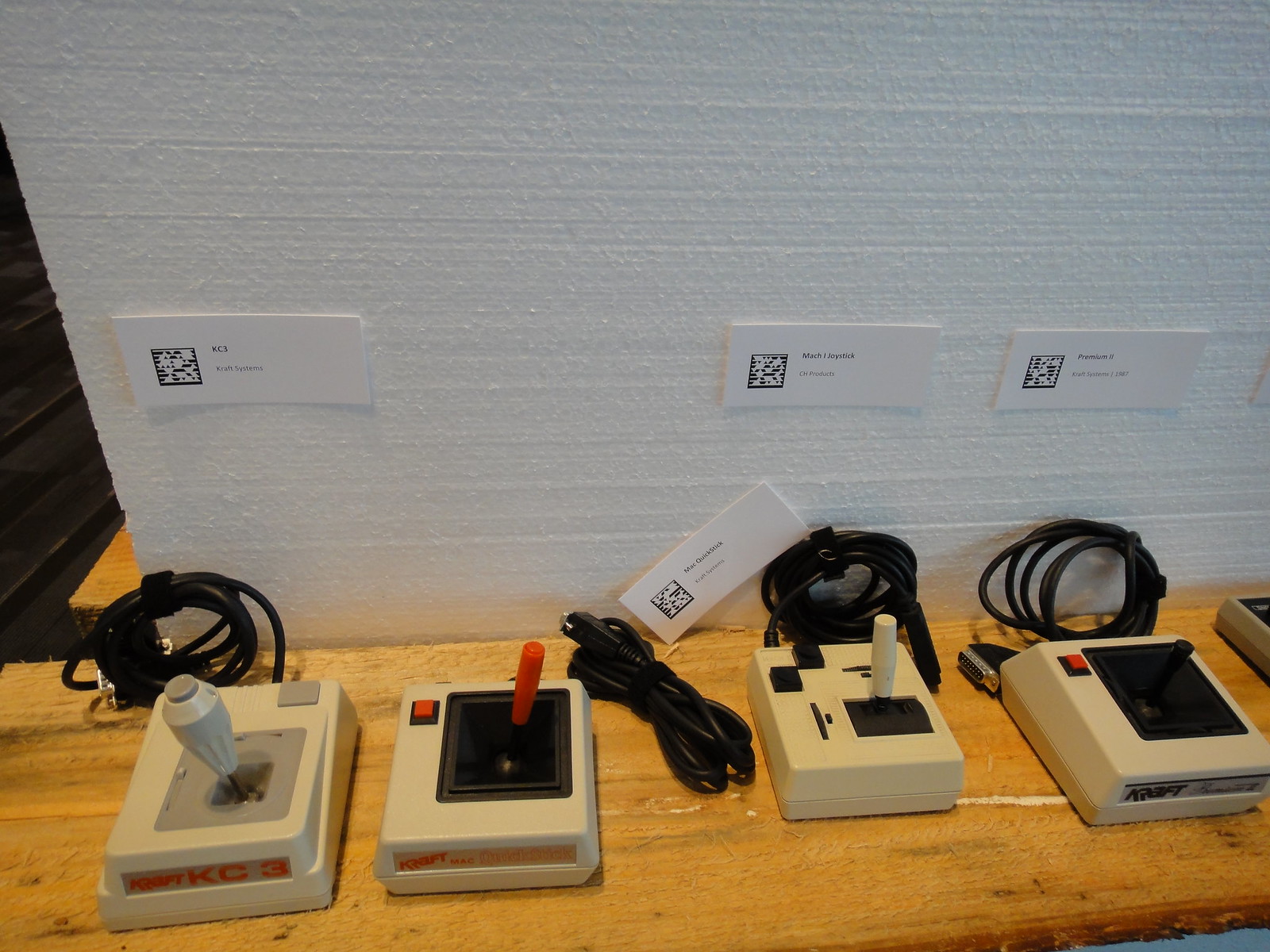The photograph captures a vintage display of old-school video game joysticks, likely set up in a marketplace or event center. The scene is shot with a wide camera, giving it an old-style appearance. The joysticks are arranged on a long, possibly homemade wooden table. Four joysticks are fully visible, with a fifth one partially off-frame to the right. Each joystick rests on a bulky, square base, with cables extending from them. The designs vary: one joystick has a silver button in the top right corner and a central handle, another features a prominent red nozzle, while a similar model has a black joystick and red button. There's also a joystick with multiple black buttons and a thicker handle.

The background consists of a white-painted drywall or styrofoam wall adorned with pieces of paper, some bearing barcodes and labels identifying the joysticks as products of the Craft brand, often labeled as "Craft Systems" or "Craft KC." The photo is rich with the nostalgic aesthetic of 1980s gaming equipment, emphasizing the taupe and beige color scheme typical of the era.